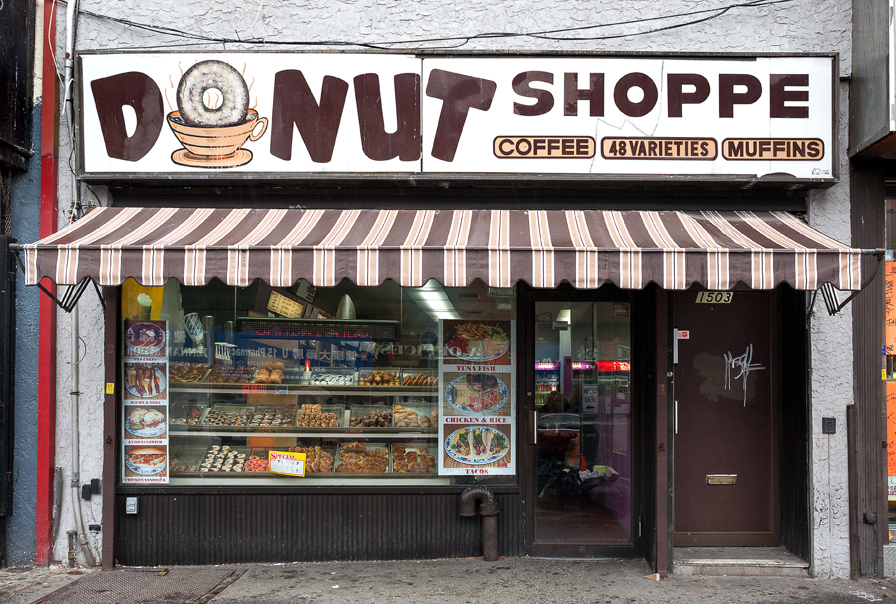This image captures the exterior of a quaint donut shop located in a slightly rundown area, indicated by the graffiti on the adjacent door and the worn condition of the sidewalk made of regular gray concrete. The shop's facade features a prominent white sign with dark brown edges reading "Donut Shoppe," where the 'O' in 'Donut' is creatively depicted as a chocolate donut with white frosting being dipped into a beige coffee cup. Below the primary sign are beige boxes with brown letters advertising "Coffee," "48 varieties," and "Muffins." The entire frontage is trimmed in brown wood, adding to the shop's cozy ambiance.

Beneath the sign, a brown-striped awning extends above a large picture window and two doors. The window prominently displays three shelves of assorted donuts and baked goods, including some savory options like tacos, chicken and rice, and tuna fish sandwiches, though the latter items are somewhat hard to make out. To the right of the window is a glass door framed in brown, leading into the shop, and to the right of this door is another brown door marked with the number "1503" at the top. The overall composition of the image suggests a warm, inviting, albeit slightly weathered, neighborhood donut shop with a rich variety of offerings.